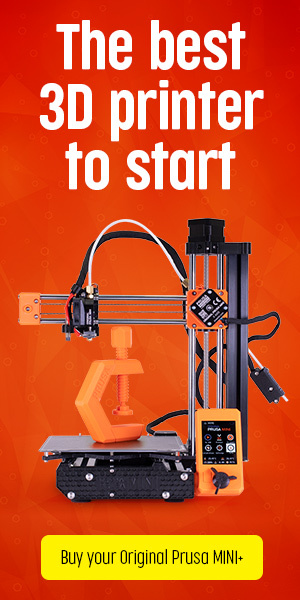The image showcases a Mini Plus 3D printer prominently in the center, accompanied by the tagline "The best 3D printer to start" at the top. The 3D printer itself is displayed with intricate detail, featuring a sleek, compact design. At the bottom of the printer, there is a black platform equipped with hexagonal screws, providing stability and support.

On the right side of the image, there is an orange device resembling a smartphone, complete with a touch screen displaying various icons. Adjacent to the screen, a twistable dial is connected to a tall structure. This structure includes three vertical pipes, each adorned with attachments and a horizontal bar extending from the top. The 3D printer is mounted on this bar, with several cables extending from it, indicating their functional role in the operation of the printer.

At the center of the printer’s platform, an orange, twisted shape is being printed, suggesting an ongoing project. The platform appears to be elevated, emphasizing the precision and capability of the 3D printer in creating complex objects.